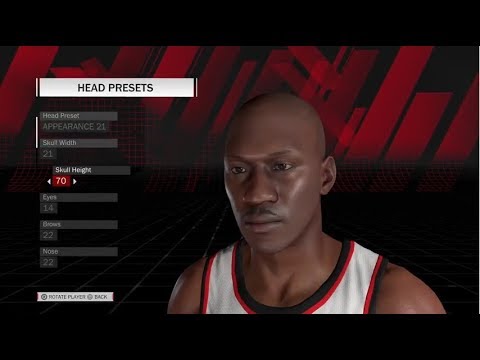Screen capture from a gaming application. The image showcases a rectangular black frame containing an animated depiction of a basketball player set against a red and black background. The basketball player, a bald-headed Black man, is displayed from head to chest. He is wearing a white basketball jersey adorned with red and black trim around the neck and armholes. To the left of the player, various game parameters are displayed. At the top of this section, "Head Presets" is clearly written in black text on a white rectangular box. Below this label, additional parameters are listed on gray rectangular bars, although the faint white text makes them difficult to read.